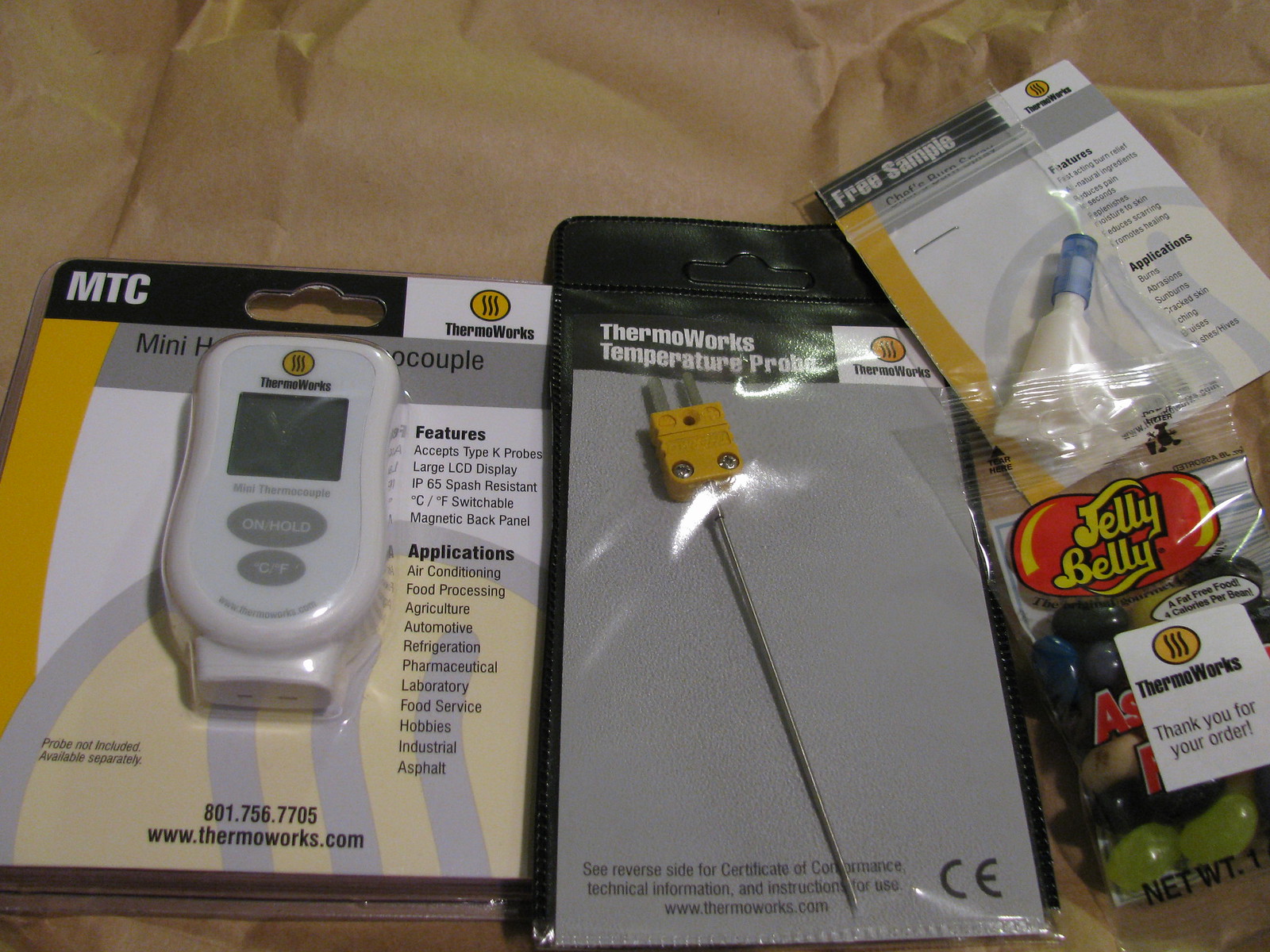This image displays a collection of four items laid out on a brown paper surface, all in their original packaging. On the left side, there is a blister plastic package featuring a white, rectangular device with a display screen and two buttons labeled "on/hold" and "Celsius/Fahrenheit." The packaging is marked with the ThermoWorks logo and the text "Mini Thermocouple." 

Next to it, in the center, there is a black package with a clear window revealing a metal probe. This packaging also bears the ThermoWorks logo and the text "Temperature Probe." The probe itself consists of a yellow main sensor part with a long metal needle extending from it. 

In the upper right corner of the image, there is a small white tube with a blue cap labeled "Free Sample Chef's Burn Spray," intended for treating burns. 

Finally, situated in the lower right corner is a bag of Jelly Belly jelly beans, featuring the ThermoWorks logo and the text "Thank you for your order." Each item stands out against the brown paper background, demonstrating a range of products associated with ThermoWorks branding.